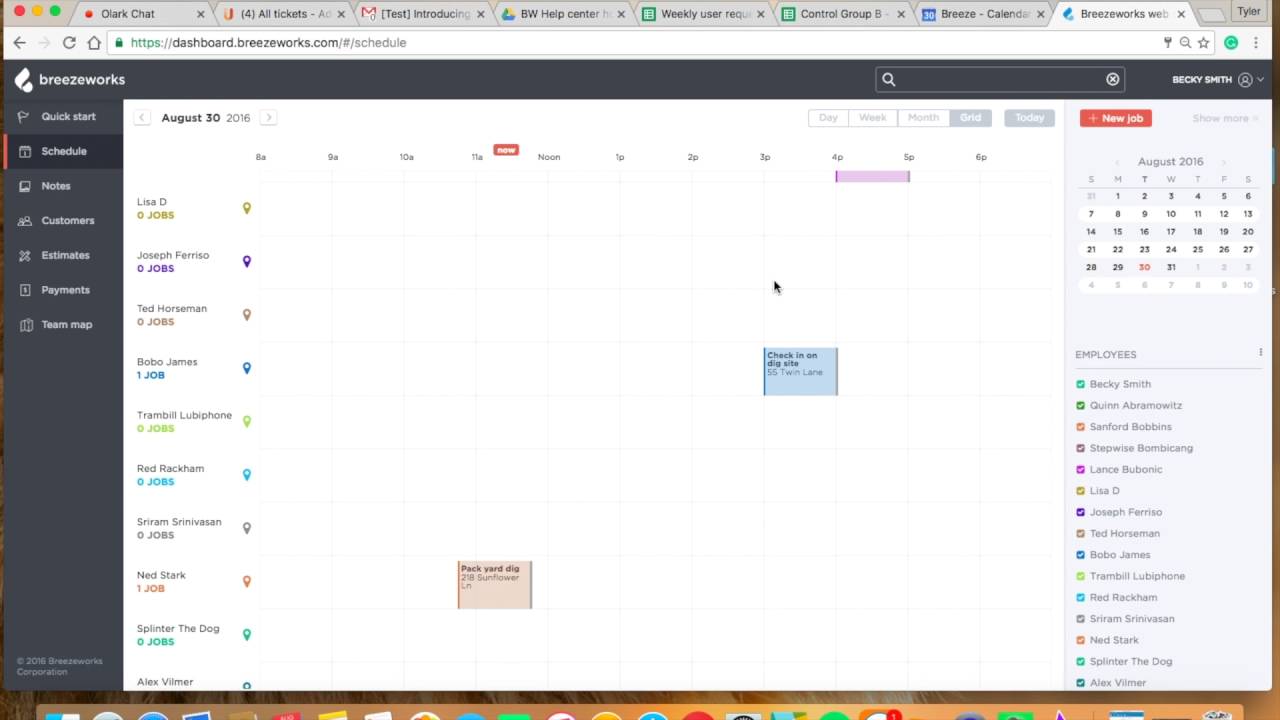A detailed screenshot of a Mac interface showcases a user’s workspace. In the top-left corner, the Mac OS title bar features three colored circles: red, yellow, and green, used for window control. Below this, a lighter gray area is populated with multiple open tabs. The address bar is white with black, unreadable text.

On the left side of the screen, against a black background, the word "Breezeworks" stands out in white at the top. A vertical sidebar lists the following options in sequential order: Quick Start, Schedule, Notes, Customers, Estimates, Payments, and an unclear term that could be "Schema Maps" or "Term Maps." Small, faint text appears at the bottom left of the sidebar.

The main section of the interface on the right is dominated by a calendar view. The date "August 30, 2016" is visible with rows beneath it listing names and schedule details, including names like “Wednesday D,” “Joseph,” and “Ted,” followed by other unreadable entries. Horizontal segments display dates, while various entries in gray blocks show scheduled activities for different individuals. Additionally, a red rectangle with white text, though unreadable, appears on the right side of the screen.

Further down, a calendar for August 2016 is prominent. There is also a sidebar containing a list of employees, distinguishable through a mix of colored indicators—reds, blues, greens, and yellows—alongside unreadable text.